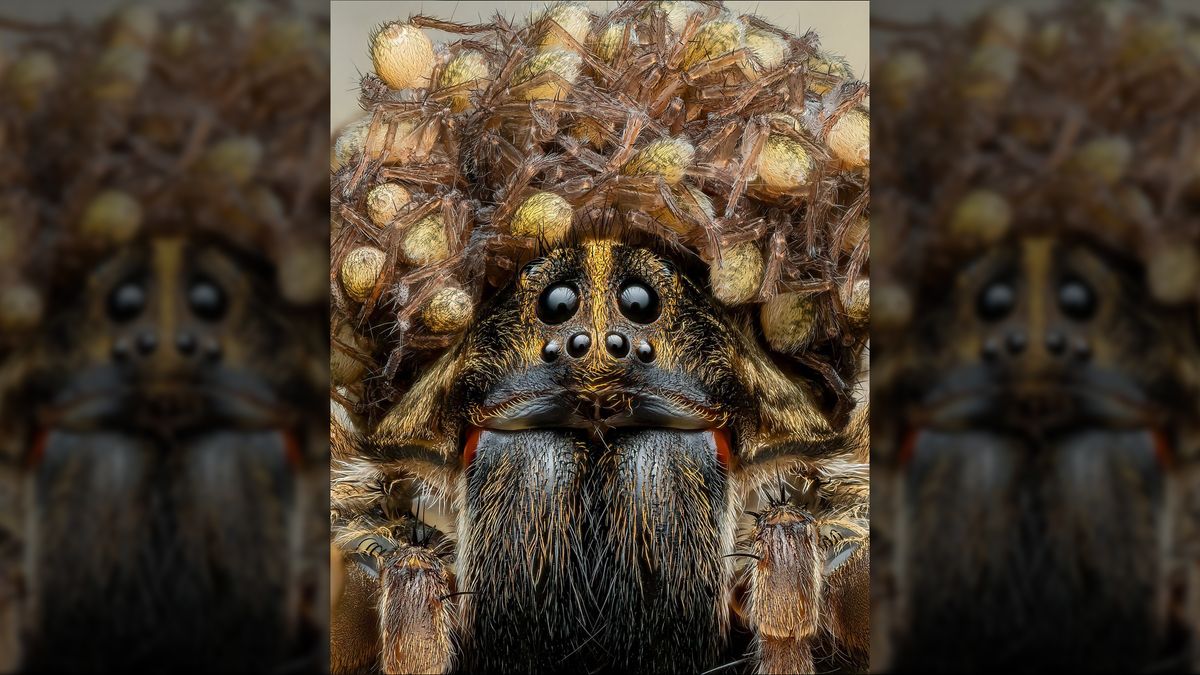This close-up photograph captures a detailed front view of a wolf spider, specifically showcasing its distinctive facial features and the brood of spiderlings clustered on its back. The wolf spider prominently displays two large black beaded eyes at the center of its face, flanked by four smaller black eyes positioned below them, giving it a total of six eyes. The spider's face is also characterized by long, hairy fangs adjacent to its first pair of legs. Its body and legs are covered in a mix of brown and black fur, with spiky hairs adding to its menacing appearance. 

A particularly noteworthy and somewhat unsettling aspect of the image is the presence of numerous baby spiders, or spiderlings, riding on the mother's back. These spiderlings have smooth, yellowish bodies and translucent legs, gathered tightly in a protective cluster. Although only a portion of the spider's face and the mass of its offspring are visible, it is clear that there are at least a dozen, if not more, spiderlings. The photograph is part of a set, showing the same image from different perspectives, highlighting the intricate details and the natural behavior of the wolf spider as it carries its young.